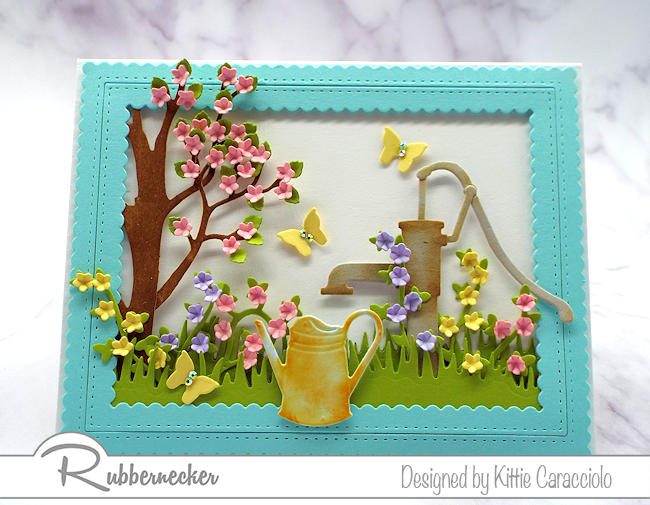This detailed color photograph captures a beautifully intricate, three-dimensional paper art piece by Rubbernecker, designed by Kitty Caracciolo. The piece is laid on a very light marble countertop. Dominating the artwork is a light bluish-teal scalloped frame with detailed stitching-like scorings, giving it an elegant handcrafted appearance. Inside the frame, we see a charming pastoral scene with various elements.

In the center foreground, an inviting light yellow watering can is depicted, seemingly being filled by an antique hand pump, colored in subdued grays and browns. The foreground is lush with bright kelly green grass, interspersed with a medley of vibrant blossoms in purple, pink, and yellow. Towards the left side, a tree with a sturdy brown trunk is adorned with delicate cherry blossoms in shades of pink and dotted with fresh green leaves. This tree's branches extend gracefully beyond the frame's border, enhancing the 3D effect of the piece.

In the upper right, three small, vibrant yellow butterflies with tiny diamond-shaped bodies flit around, adding to the scene's liveliness. The three-dimensional butterflies and several blossoms extend past the confines of the frame, further amplifying the depth and realism of the artwork.

Significantly, the bottom of the piece bears the grey script inscription "Rubbernecker," alongside the credit "designed by Kitty Caracciolo," affirming the creators' meticulous craftsmanship and distinctive design. This art piece stands out as both a decorative item and a captivating testament to detailed paper artistry.